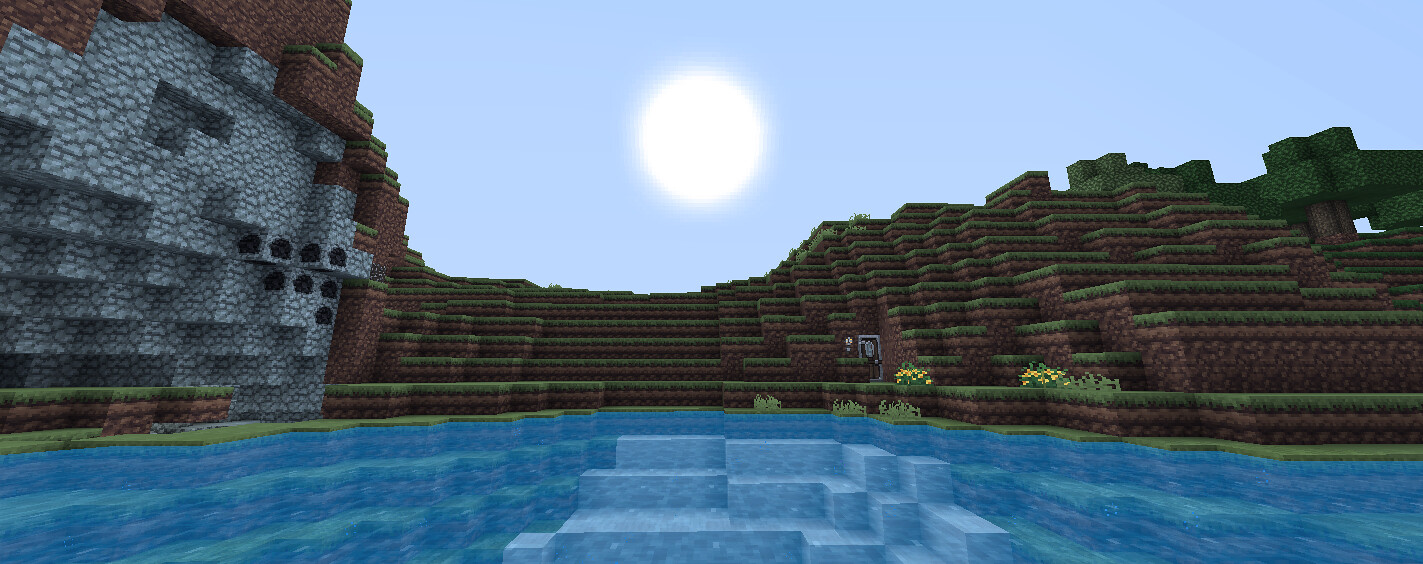This is a detailed screenshot from the popular game Minecraft. The entire scene is composed of variously colored and textured blocks, reminiscent of a digital Lego landscape. In the foreground, there's a clear blue body of water, transparent enough to reveal the blocky terrain of the lake bed or riverbed underneath. This water is rendered with different shades of blue blocks, creating a sense of depth.

The middle section of the image features a series of tiered, stair-like layers made of blocks that resemble an amphitheater or terrace. These steps transition from what appear to be marble-like blocks to grassy areas, and finally to brown and gray brick steps. To the left, there is a distinct rocky cliff face, illustrating the in-game world's native block structure.

In the upper portion of the screenshot, the landscape rises into mountainous terrain with blocks simulating dirt, rock, and grass. The entire scene is uniformly made up of geometric chunks—the hallmark of Minecraft's aesthetic. Prominently, in the center of the upper half, there's a bright white sun set against a very light blue sky, casting light onto the landscape. Additionally, a couple of yellow flowers, perhaps marigolds, dot the right side of the image, adding a touch of color to the earthy palette.